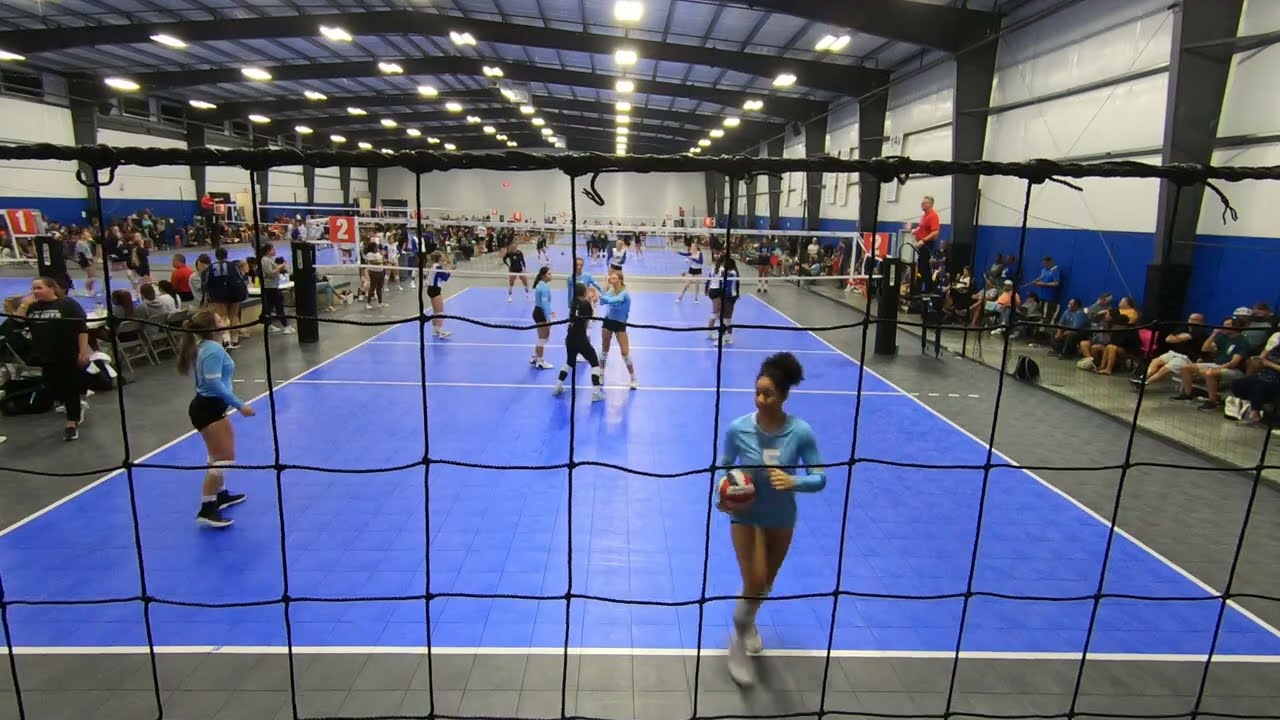This horizontally-aligned rectangular image captures an indoor volleyball game set in a spacious gymnasium. The scene is illuminated by numerous fluorescent lights affixed to the high ceiling, casting a bright glow over the entire area. The upper walls are white, while the lower sections sport a blue color. The game's focal point is a white net dividing the court, which features blue flooring with white boundary lines and is surrounded by gray tiles.

In the foreground, high school girls’ volleyball teams are in action. The team visible on our side of the net wears blue long-sleeve jerseys and short black shorts, whereas the opposing side—though blurred—can be identified by their black shirts and blue shorts. A girl on the right, holding a volleyball and seemingly preparing to serve, approaches the net.

Spectators, lacking bleachers, are scattered around the court, seated casually in chairs. The gym’s layout suggests it's hosting a tournament, as multiple courts are visible—one in the distance and more blue courts discernible in the upper left corner. The presence of many courts, coupled with chairs scattered between them, highlights the busy, competitive atmosphere of the event. Various colors, including black, grey, white, blue, red, yellow, orange, and tan, are evident across the scene, hinting at the diverse elements present in this lively sporting environment.